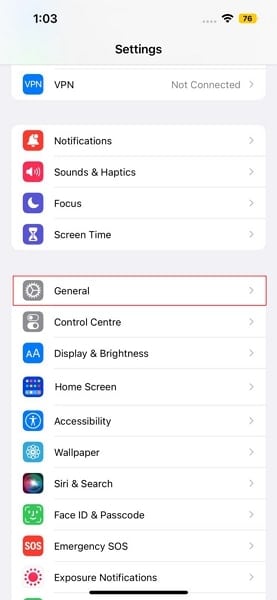The image is a screenshot of a smartphone’s settings menu. 

In the top left corner, the time is displayed as 1:03. The top right corner shows signal strength represented by four light gray dots, a fully filled black Wi-Fi icon, and a battery icon at 76%, colored yellow. 

Centered below the status bar, the word "SETTINGS" is prominently displayed in capital letters. The menu options are organized into distinct sections. 

The first category includes 'VPN', with an accompanying icon to the left and labeled as "Not Connected" with an arrow pointing to the right, indicating additional options.

Further down, there is a 'Notifications' section subdivided into individual options such as Sounds & Haptics, Focus, and Screen Time. 

Below this section, a longer box provides additional settings which include, but are not limited to:
- General
- Control Center
- Display & Brightness
- Home Screen
- Accessibility
- Wallpaper
- Siri & Search
- Face ID & Passcode
- Emergency SOS
- Exposure Notifications

Each setting within this comprehensive list has its own icon to the left and implies a separate menu for more specific configurations.